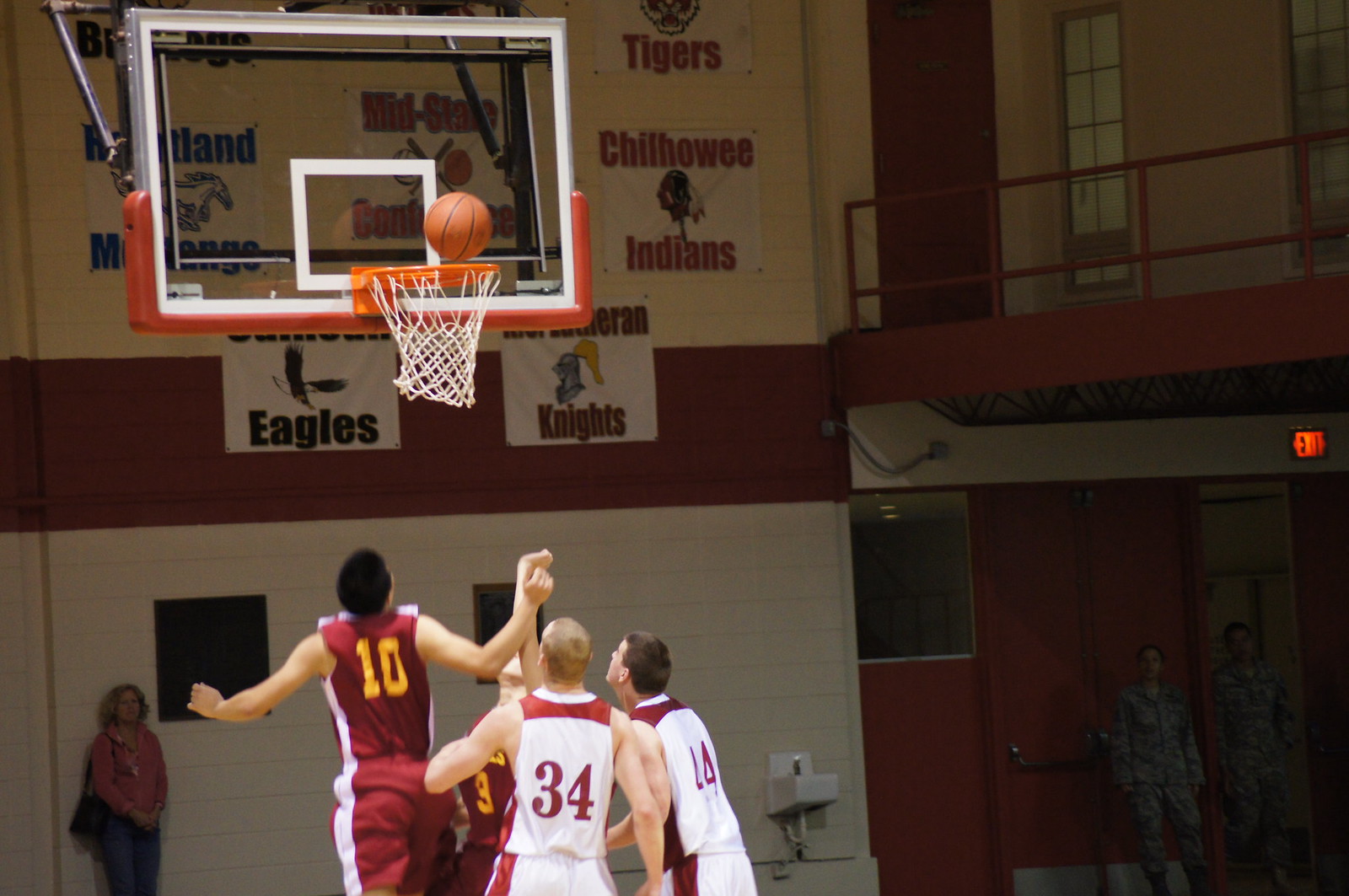This photograph captures an indoor high school basketball game in a rectangular gymnasium, wider than it is tall. In the foreground, we see the backs of four Caucasian basketball players. Two players are clad in dark red uniforms with white stripes and gold lettering, displaying the numbers 10 and 9. The other two players are in white uniforms with burgundy red accents and red numbers, showing 34 and possibly 24. All players have their attention fixed upwards, where a basketball precariously balances on the hoop's rim, suggesting an imminent score. 

Behind the players, a white brick wall painted with a red stripe and adorned with various school banners can be seen, including names like the Midland Mustangs, the Eagles, the Knights, the Chiloe Indians, and the Tigers. A woman with a handbag watches the game intently. To the far right, beneath an exit sign, stand two individuals in military uniforms near a set of red doors. Above them, a scaffolding walkway adds to the gymnasium's structural detail.